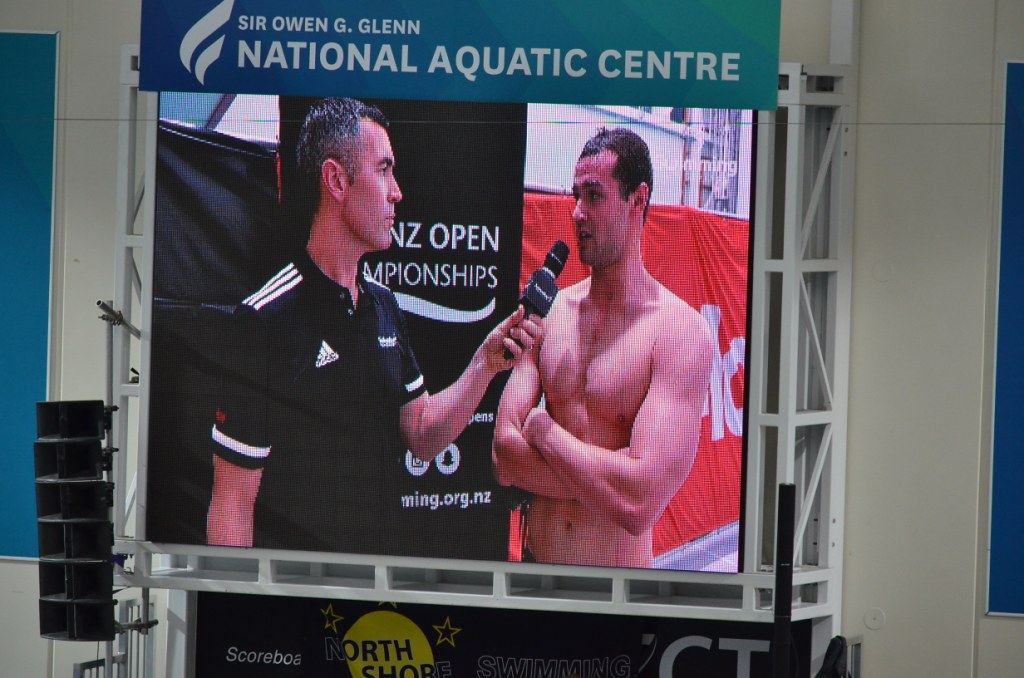The image shows a shirtless swimmer, who appears to have just exited the pool, being interviewed by a man in a black Adidas polo shirt with white stripes on the shoulders and rings around the arms. The interviewer, a slightly pepper-haired man, holds a microphone up to the swimmer, likely capturing his thoughts post-race. The scene is set against a backdrop featuring two banners: one blue banner at the top displaying "Sir Owen G. Glenn National Aquatic Center" with their logo, and another red banner to the right, partially obscured by the swimmer, with large, unreadable white lettering. The lower banner reads "Open Championships," though additional details are illegible. The image gives the impression of a post-race interview at a competitive swimming event, set at a national aquatic center.